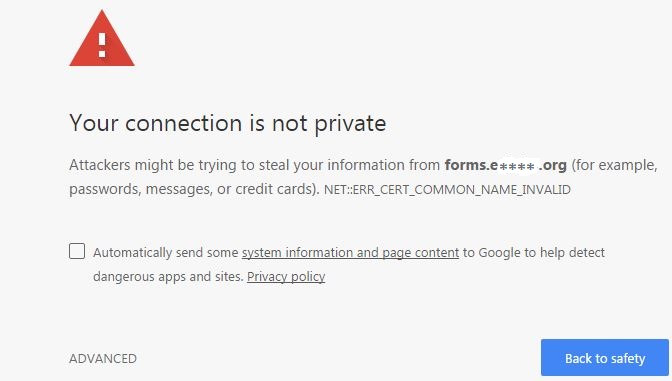The image features a light gray background and is rectangular, significantly wider than it is tall. In the top left corner stands a prominent large red triangle with an exclamation point in the middle, serving as the image's focal point. Beneath this triangle, in the largest text on the page, is the warning: "Your connection is not private. Attackers might be trying to steal your information from forms.e**.org. For example, passwords, messages, or credit cards."

Following this warning is an error message coded as: "NET::ERR_CERT_COMMON_NAME_INVALID."

Positioned towards the lower left side of the page, there is an unchecked box with the text: "Automatically send some system information and page content to Google to help detect dangerous apps and sites," with "system information and page content" underlined. Immediately below this is the phrase "Privacy policy," also underlined.

At the bottom of the page, in the lower left corner, the word "ADVANCED" is prominently displayed in all capital letters. Meanwhile, the bottom right corner features a blue rectangle with white text inside it that reads, "BACK TO SAFETY."